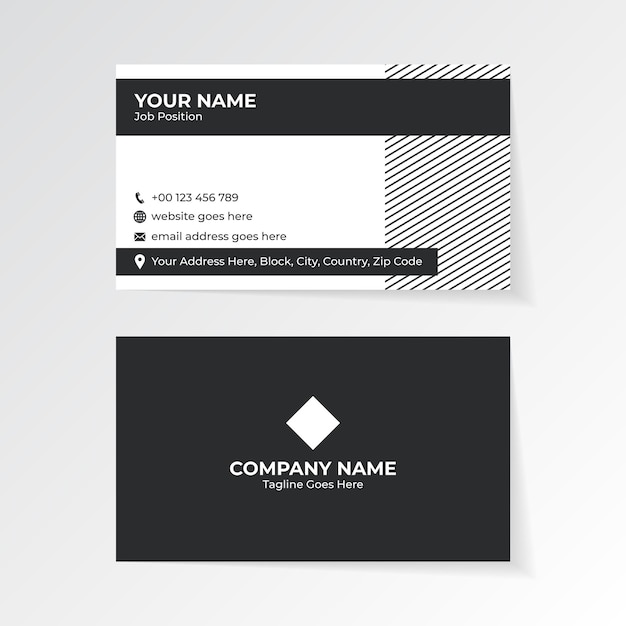This image depicts both sides of a customizable business card design against a neutral background. The back of the card is predominantly black, featuring a prominent white diamond in the center. Beneath the diamond, in clean white or grayish font, are the placeholders "company name" and "tagline goes here." The front of the card is showcased above the back, with detailed placeholders on a striking black-and-white layout. The top portion has a black band running across, displaying "your name" and "job position" in white font. Below this, a white background is adorned with diagonal black stripes on the right side, creating a dynamic design. In the middle section, icons and placeholders indicate where a phone number, website, and email address should be. Each of these fields is accompanied by respective icons: a phone, an internet globe, and an envelope. At the bottom, another black band displays "your address here," followed by fields for block, city, country, and zip code. This card design is a versatile template, allowing users to easily customize it with their own business details.